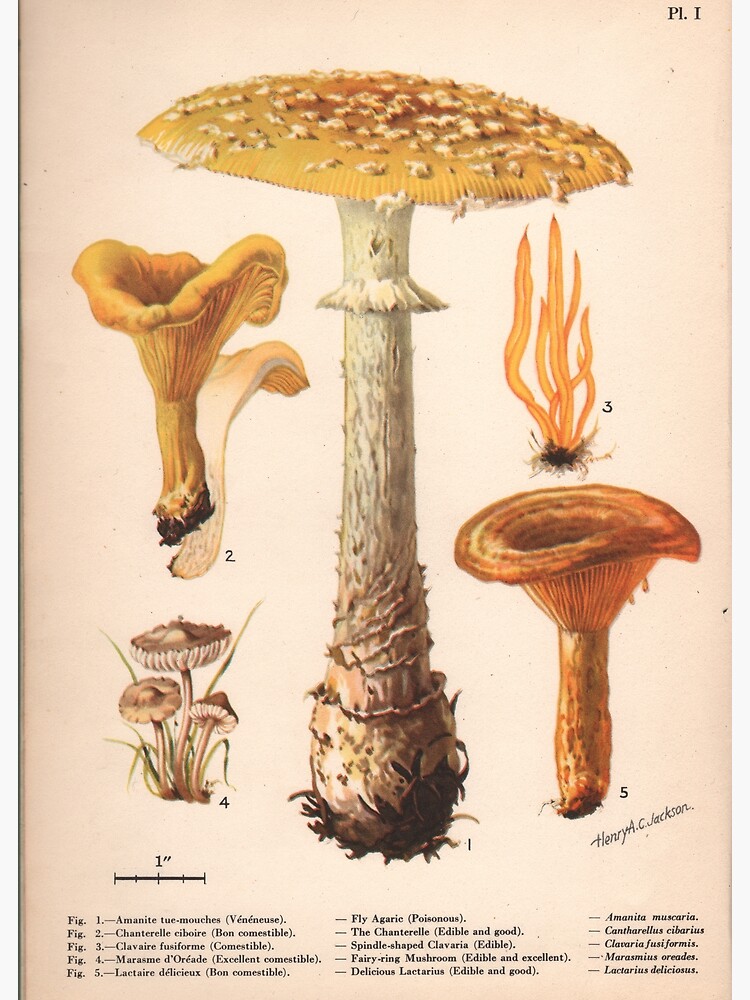This horizontally oriented image features a detailed, old-school botanical illustration of various fungi, meticulously drawn on a slightly yellowed page with darker edges. Dominating the center is a large mushroom with a tall, narrow white stem extending down to a root base. The mushroom cap is orange with beige specks and has a distinctive ring around the top of the stem. 

Surrounding the central mushroom are four smaller illustrations on either side, depicting different types of fungi. On the left, there's a mushroom resembling a blooming yellow flower, and below it, a small cluster of three beige mushrooms nestled in grass. On the right side, there's a group of long, skinny orange fungi that look like seaweed or worms, followed by a mushroom with a thick stem and a funnel-shaped cap.

Below these illustrations, a scale marker indicates that one inch equals a certain length in real life, and annotations label each figure, such as "figure one, ammonite to mucis (fly agaric, poisonous, Amanita muscaria), figure two, chanterelle (edible and good, Bon comestible)." Additionally, the signature of Henry A. C. Jackson appears in the bottom right corner. This beautiful and informative chart combines scientific accuracy with artistic flair, offering a comprehensive overview of various mushroom types.